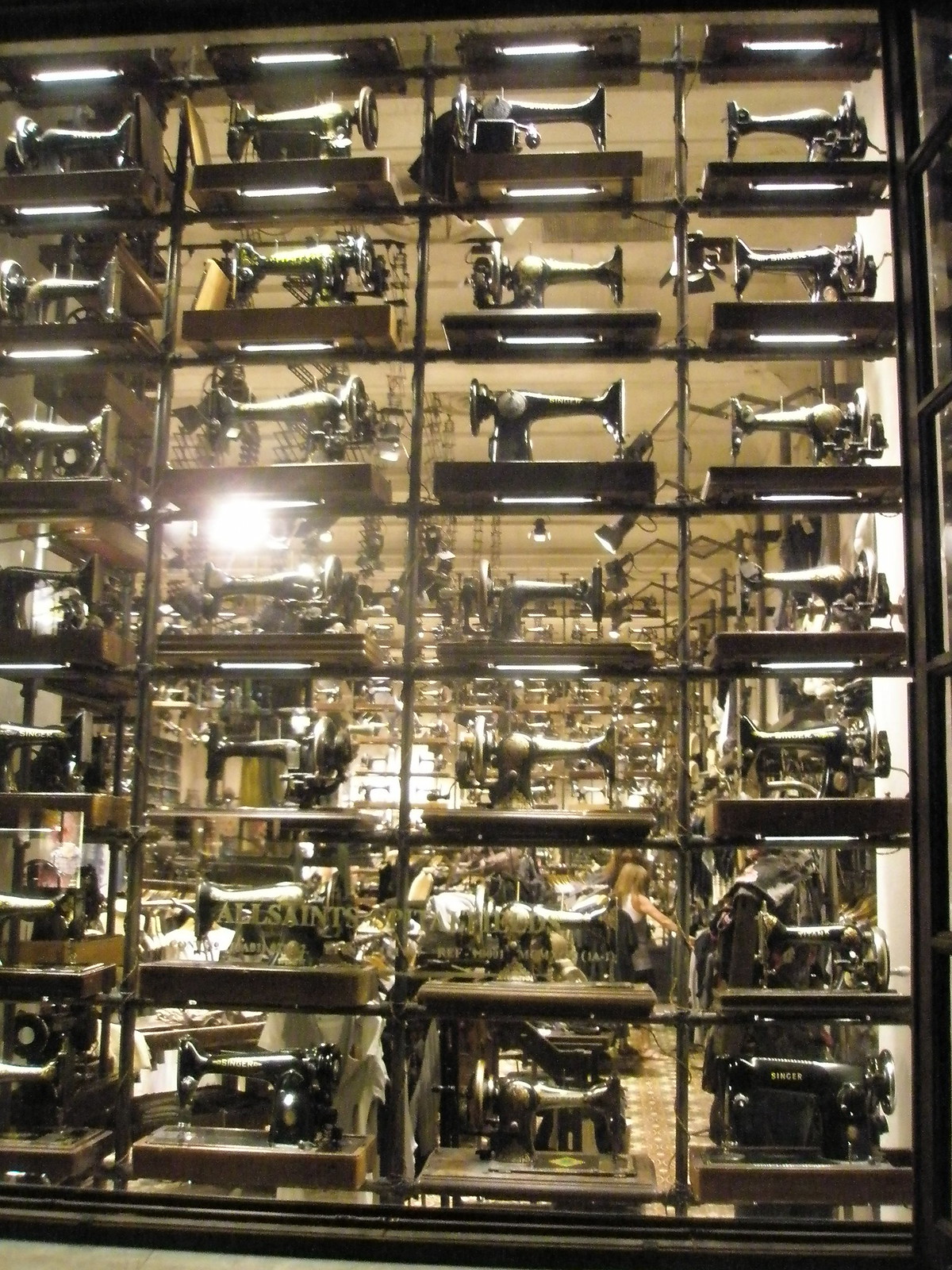This color photograph, taken in portrait format, showcases the striking storefront of All Saints Spitalfields in London. The store's front display case, constructed from metal and glass, features a meticulously arranged collection of antique Singer sewing machines. These vintage machines, adorned in hues of black, gold, and silver, are neatly stacked eight to nine high and four across on brown shelves. The glass window bears gold lettering that reads "All Saints." Though not a dedicated sewing machine store, the high-ceilinged, two-story interior hints at a space possibly used for clothing merchandise. Behind the display, a well-lit room filled with other machinery and a possible workspace is partially visible.